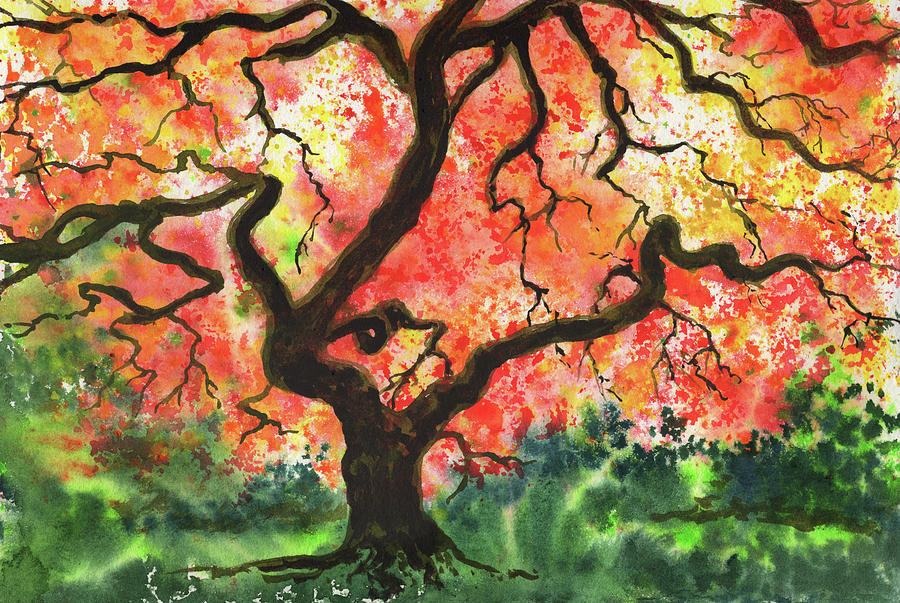This painting portrays a solitary, prominent tree with a thick, brown trunk displaying numerous gnarled and sprawling branches. The tree stands rooted in a lush, green lawn that forms the base of the composition. Its branches extend in various directions, creating an intricate network of limbs, with one particularly distinct branch shaped like a human eye near the center. The foliage is an impressive array of vibrant red, orange, and yellow leaves, interspersed with green splotches that add depth and contrast to the scene. The leaves are distributed throughout the canopy and even appear as splotches in the sky, enhancing the uniqueness of the artwork. This detailed and vividly painted tree dominates the scene, making it a visually striking and intricate piece.